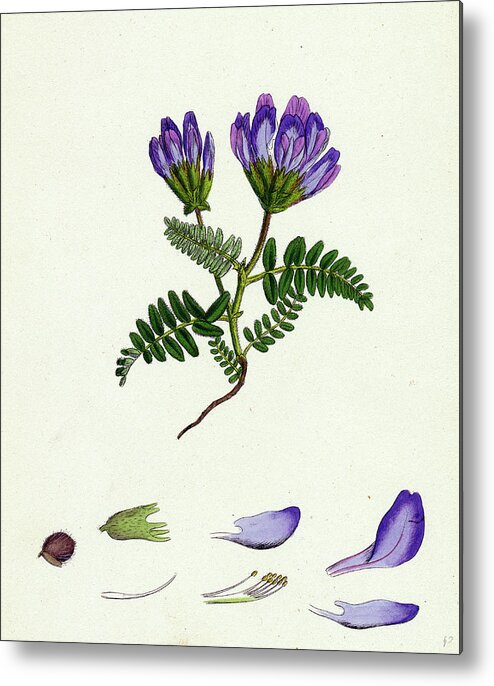This image showcases a framed illustration against a cream-colored background, suitable for hanging on a wall. It features two purple flowers with petals in varying shades of violet, lavender, and pink, attached to green stems with fern-like, pennelia leaves. The flowers' petals are primarily purple with some green at their base. Below the blooms, the flower has been deconstructed showing individual parts: a brown acorn-like seed, three distinct purple petals, a single stamen, a cluster of stamens, and a green base where the petals attach to the stem. Details of the petals reveal different development stages from the flower. There is text at the bottom of the image, but it is unreadable. This botanical illustration combines elements of scientific documentation and aesthetic presentation reminiscent of Audubon's style.